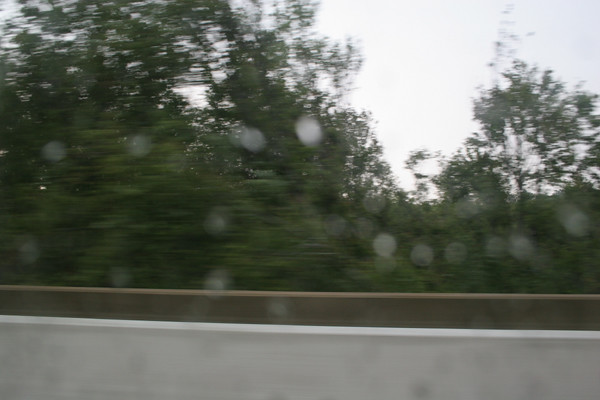A photograph captures a tranquil, rainy scene viewed through a window adorned with delicate raindrops. The sky is overcast, casting a diffuse, whitish light across the landscape. In the foreground stands a low, light-gray cement wall, topped with a brown railing. Beyond the wall, the tops of lush green trees peek into view, suggesting a significant drop in elevation on the opposite side of the railing, further emphasizing the sense of depth in the scene. The overall atmosphere is one of calm and contemplative serenity, accentuated by the muted, cloudy light and the gentle presence of the rain.